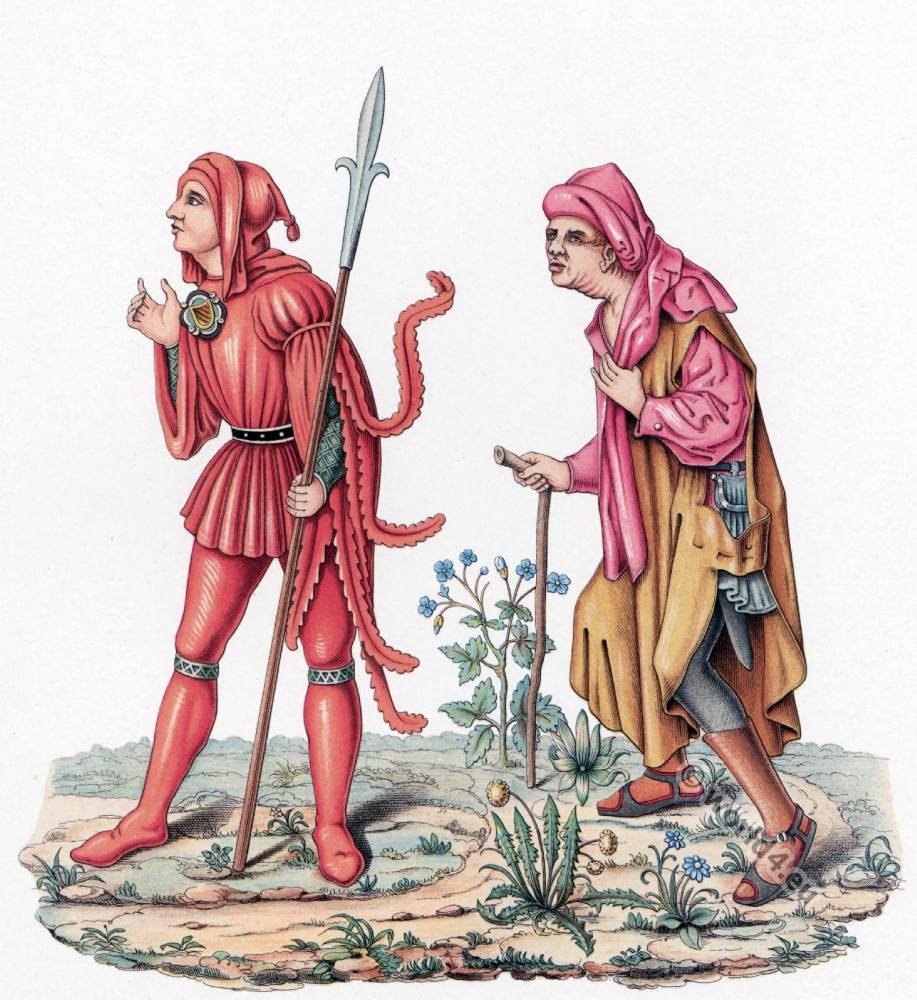This vertically rectangular full-color print features a detailed depiction of two figures dressed in Middle Ages or Renaissance attire, set against a very faint off-white, light-gray background. The ground at the bottom is brown dirt interspersed with green grass, plants, and flowers, including dandelions and blue blossoms.

The figure on the left, likely a man, is dressed entirely in red. He wears a red tunic with puffy sleeves and red leggings accompanied by white shoes and white stockings. Around each knee is a black band with silver zigzag patterns. He sports a red hood, and a black belt with some kind of ornamentation fastened to his chest. His left sleeve is divided into streamer-like strips, some of which appear to be blowing in the wind. In his left hand, he firmly grasps a wooden spear with a distinctive metal tip, featuring two curled metal parts that rise to a point in the center. His right arm is bent upward towards his face, as if he's attempting to pinch something.

The figure on the right, whose gender is ambiguous, leans slightly forward and uses a walking stick with a bent top as a handle. This figure wears black sandals, grey or greenish pants, and a yellowish robe over a pinkish shirt. They have a pink scarf or headband and are characterized by an ample amount of folds or wrinkles around their neck. Both figures are facing to the left, absorbed in a scene that emphasizes the historical and artistic richness of the era. At the bottom of the print, a diagonal strip bears the text "copyright world for .eu".